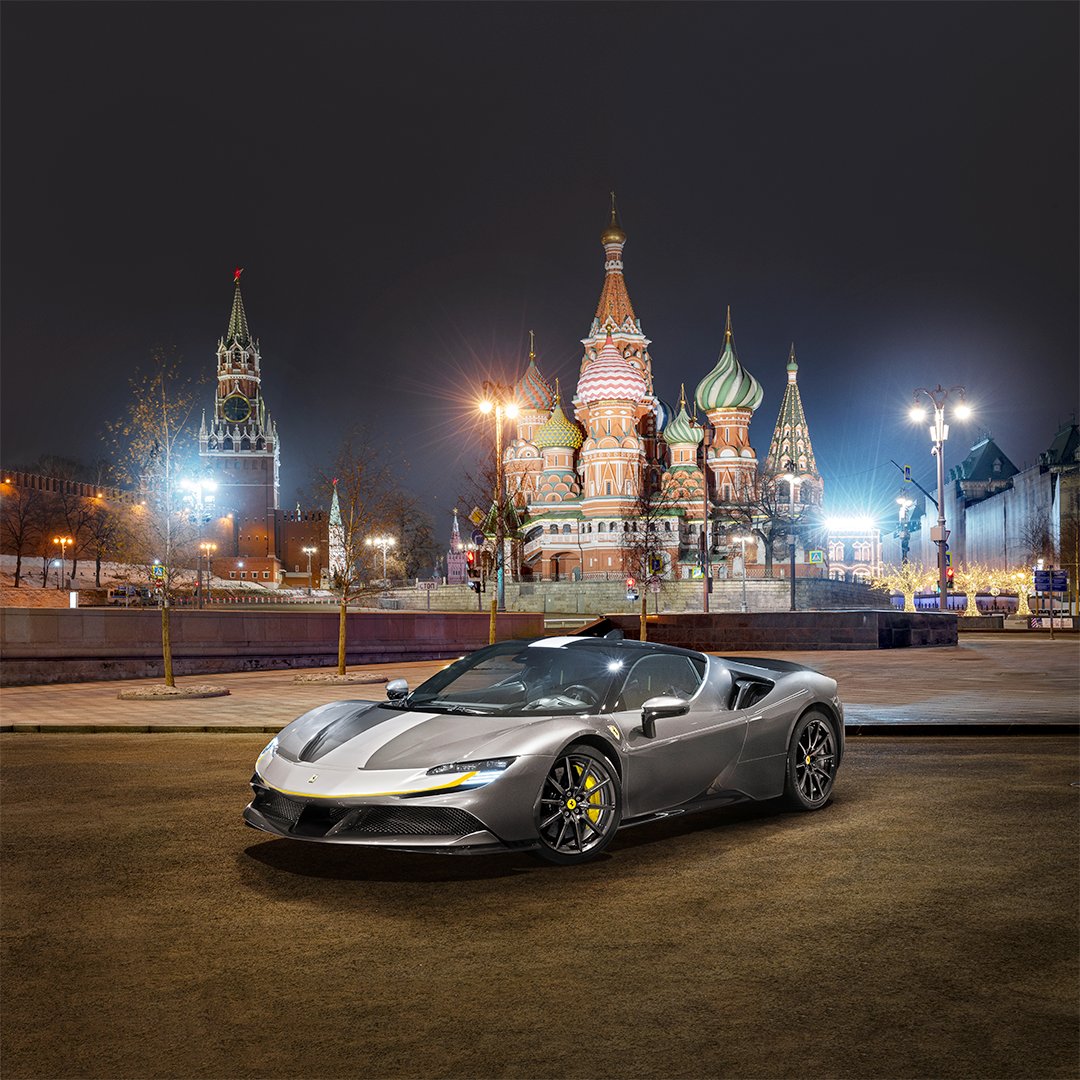The image depicts a nighttime scene in what appears to be a Russian city, featuring an iconic castle-like building in the background. The sky is very dark, suggesting either heavy cloud cover or very late evening. The castle has intricate details with a central tower capped by a spire, and several smaller towers with distinct green roofs, some spiraling with patterns. To the left of the castle stands a large brown clock tower, its faces illuminated.

The foreground is dominated by a sleek, expensive sports car, appearing to be either a Porsche or a Lamborghini, striking in its highly-reflective silver color with a black rooftop adorned by a white stripe. The car's front end looks aggressive, with a mix of white and black features, and its silver rims with yellow trim enhance its sporty appearance. Despite the dimly lit sky, the scene is well-lit by numerous streetlights and lamps, which highlight the car and the detailed architecture in the background. The ground appears to be a stone or concrete slab, possibly lined with AstroTurf, and no people are present, lending a serene, secluded atmosphere to the composition.